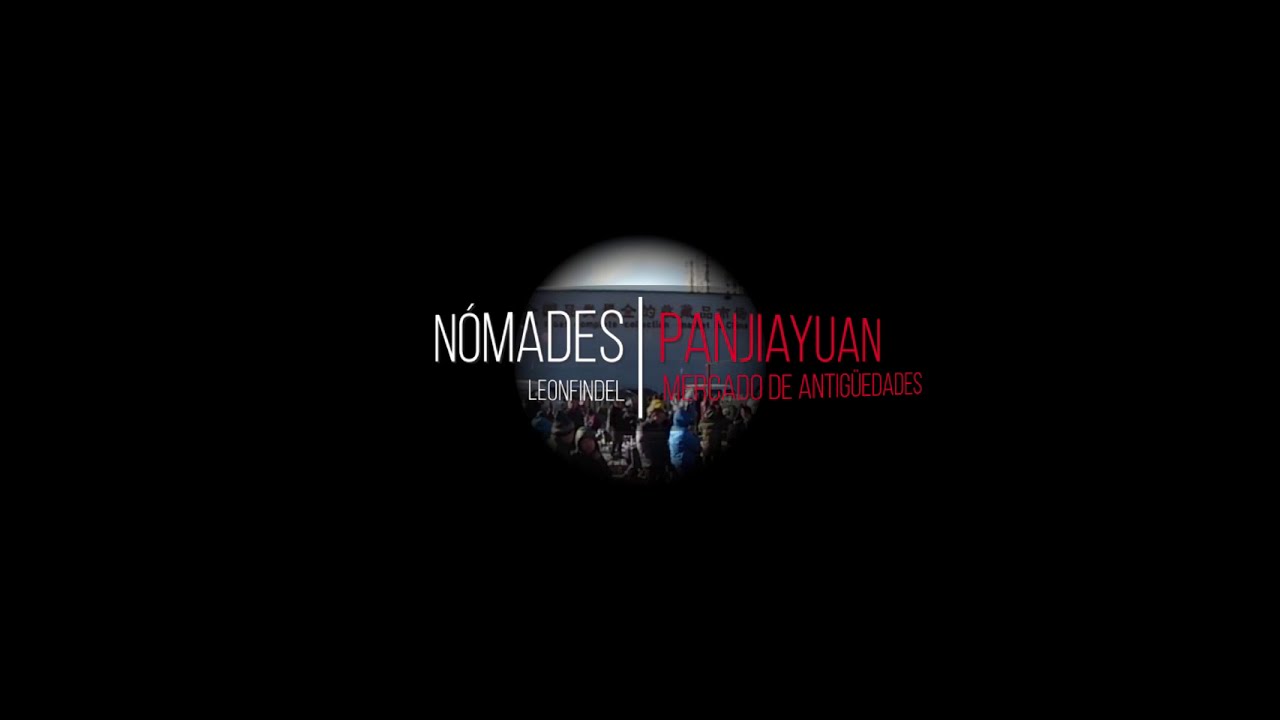The image appears to be a poster with a predominantly black background featuring a central circular photo of a warmly dressed crowd, possibly at a concert or gathered outside a building, wearing hats and hoods. Over the image, bold white letters spell out "N-O-M-A-D-E-S" accompanied by the vertically aligned red letters "P-A-N-J-I-A-Y-U-A-N" in thin font. Beneath "Nomades" is the name "L-E-O-N F-I-N-D-E-L" in white, and to its right, partially obscured, is additional text in red stating "De Antigüedades." The photo has a tunnel vision effect, further emphasizing the text overlaid on the scene.